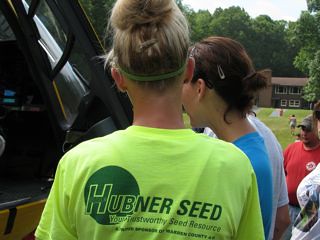In this outdoor scene, a small group of people faces away from the camera, concentrating on a barely discernible contraption or vehicle to the left. The central figure, a woman with dirty blonde hair styled in a bun, wears a bright yellow t-shirt emblazoned with green lettering that reads "Huebner Seed" with some additional, indistinct text. She sports a green band around the back of her head, near her nape. To her immediate right, another woman with her hair up and secured by a clip is visible in a blue t-shirt, though only the side of her face and neck can be seen. More people are scattered towards the right background, against a backdrop that includes a grassy area, a brown building, and a cluster of trees. In the upper right corner, the sky is partly visible, featuring shades of blue interspersed with white patches.